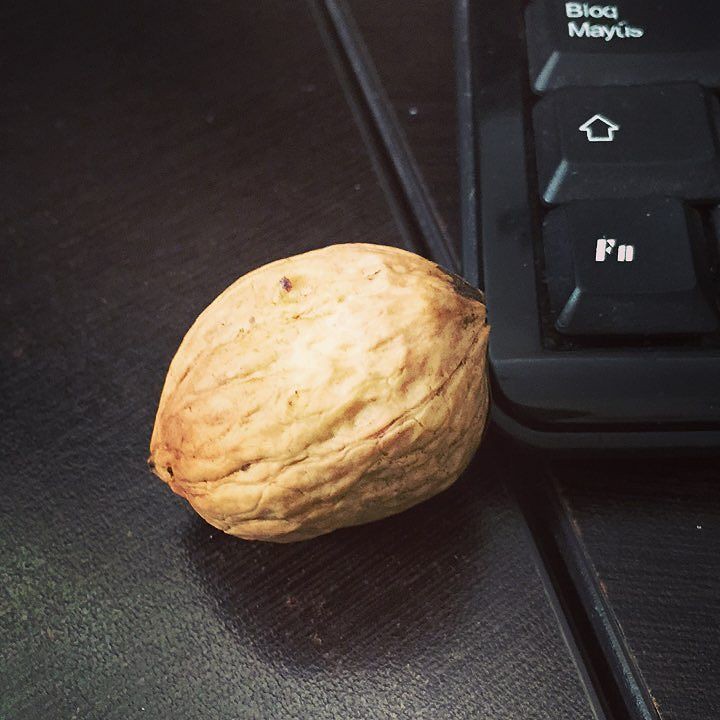The photograph captures a detailed close-up of a cracked, tan-brown walnut shell with distinct creases, pits, and grooves, sitting on a hard black surface that appears to be the junction of two tables, marked by a central crease running from the bottom right corner to the top middle of the image. Adjacent to the walnut, in the top right corner, a thin, black laptop keyboard is partially visible, showcasing three keys: 'FN' in the bottom left, an up arrow key above it, and another key with white lettering partially reading 'B-L-O-D' on the top line and 'M-A-Y-T-I-S' on the bottom line. The entire composition is set against the contrasting textures and colors of the black surface and the textured walnut shell in the center.